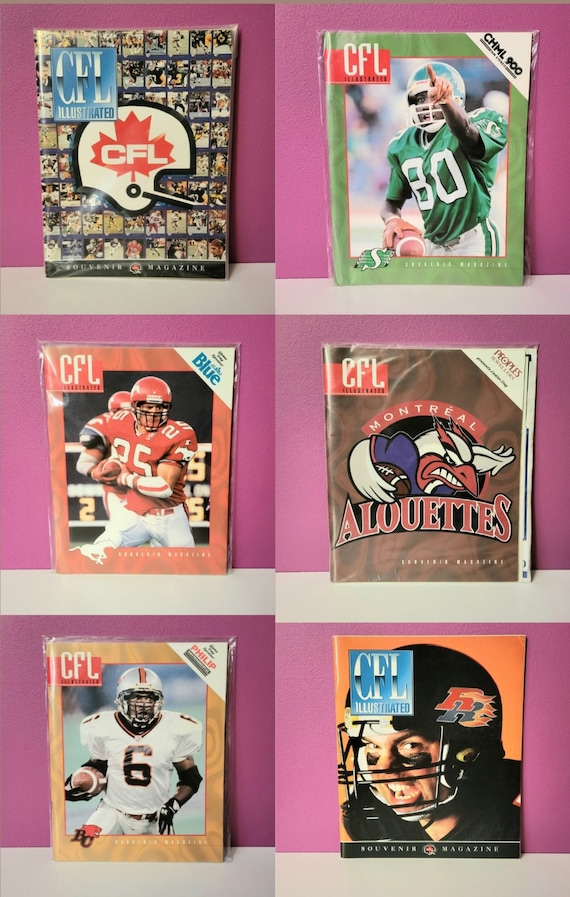The image features six distinct CFL (Canadian Football League) magazine covers arranged in two columns and three rows. Each cover showcases dynamic football-themed artwork with a consistent motif of the CFL logo and a red maple leaf emblem. The top left cover, titled "CFL Illustrated," depicts a white football helmet adorned with the CFL logo. Adjacent to it, the top right cover features a football player in a green helmet and jersey (number 80) making a number one hand gesture while holding a football. The middle left cover highlights a player in a red jersey (number 85) ready to throw a football, while the middle right cover illustrates an angry bird holding a football with "Montreal" emblazoned above. The bottom left cover presents a player in a dark jersey (number 6) carrying a football, and the bottom right cover solely displays the head of a football player with sport markings on his cheeks, grinning widely. The left side of the arrangement exudes darker hues like deep purple, whereas the right side leans towards pinkish and greenish tones, giving each column a distinct thematic appearance.